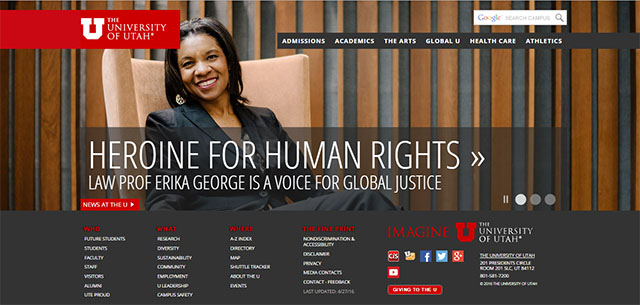A professional portrait prominently featured on the University of Utah website showcases an elegant African American woman in a suit, who appears to be approximately 34 years old. She sits confidently in a large chair, her straight black hair framing her smiling face. Accompanied by the title "Heroine for Human Rights," this image highlights Law Professor Erica George as a dedicated advocate for global justice. The webpage offers various navigation options, including Admissions, Academics, The Arts, Global U, Health Care, and Athletics, and features a red and white "News at the U" button. In the upper right corner, there is a Google search bar, and links to social media platforms like Facebook, Twitter, and Google Plus, providing multiple avenues for community engagement and information.